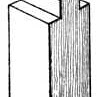The image is a very small, likely computerized or hand-drawn, sketch with 3D rectangular shapes resembling wooden pieces. The background is entirely white, with black lines creating the 3D effect. In the foreground, there is a rectangular block that stands vertically, resembling a 2x4 piece of wood. The top of this block features a narrow horizontal rectangle, and two longer lines extend downward from it, giving the impression of it standing upright.

On the right side, the image includes vertical lines, almost pencil-width, that start from the end of the main rectangle and extend downwards. This right section is more detailed with shading, suggesting wood grain. The main block appears to be shaded and textured to mimic the appearance of wood, enhancing the three-dimensional look. Additionally, a white triangle is visible in the upper right corner of the image, adding a bit more dimensionality and contrast. Overall, the image focuses on portraying a piece of wood with shaded and textured details, set against a minimalistic white background.